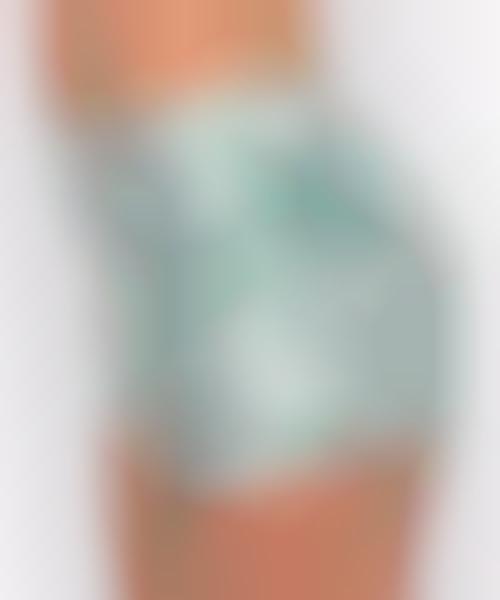The image is a completely blurred abstract composition with no discernible object. The top and bottom parts of the image exhibit an orange to pinkish hue, while the central section is predominantly green with blue undertones. The green area, which occupies the majority of the image, starts darker near the top and transitions to lighter shades towards the bottom. This central section has a slight bend towards the top left before straightening in the middle. The colors are not uniform, particularly in the green section. The background of the image, especially on the left and right edges, appears white. The overall effect is akin to viewing something with poor vision, entirely out of focus, potentially reminiscent of a piece of abstract art. The indistinct nature and the blending of colors might vaguely suggest a leg with a knee brace, but this interpretation remains highly speculative due to the extreme blur of the image.